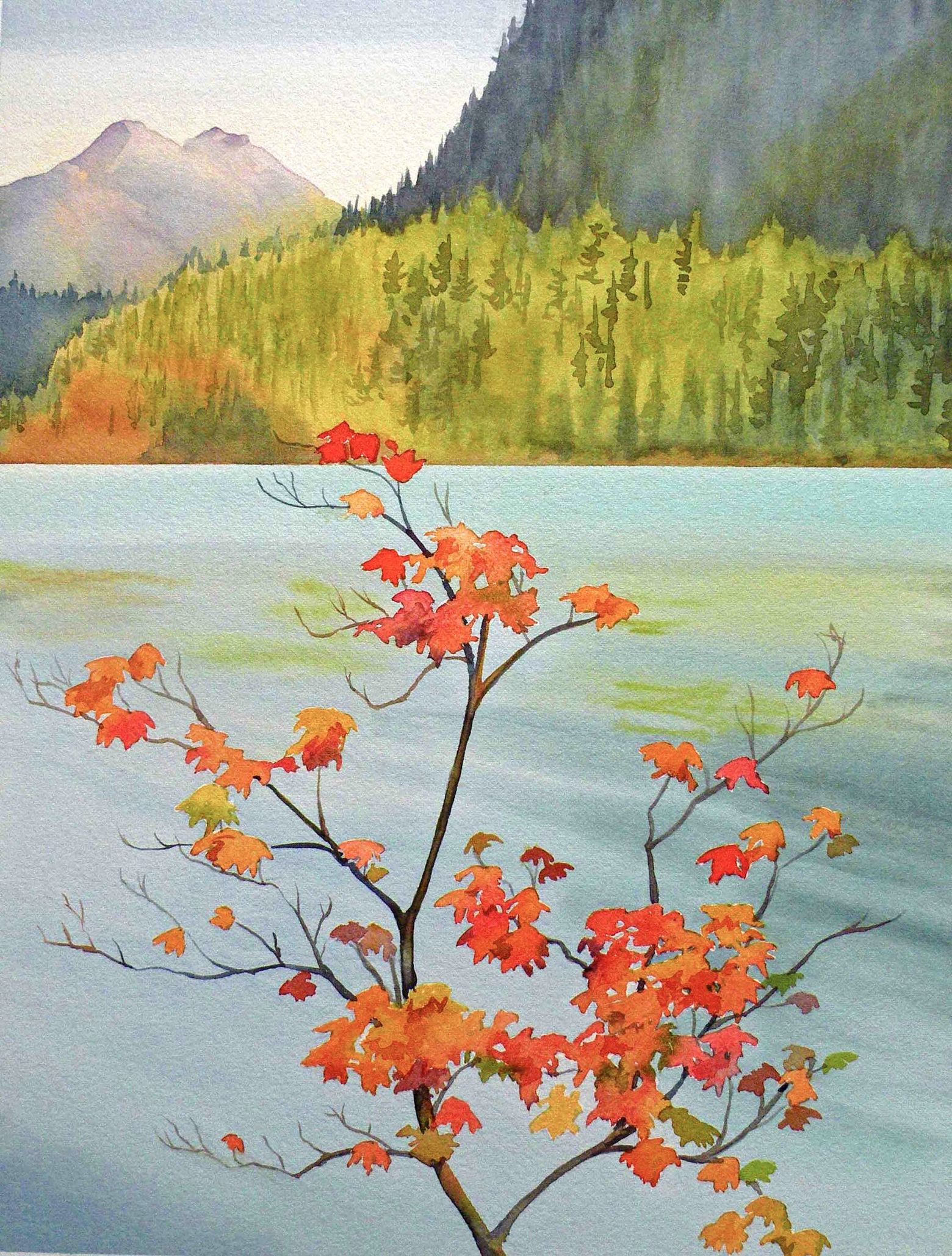This vertically oriented, full-color painting captures a serene, daytime nature scene set in autumn. Dominating the foreground, slender brown branches adorned with a sporadic array of vibrant reddish-orange and a few lingering green leaves spread outwards, reaching nearly to the edges of the image. They rise from the bottom center and splay outward, almost disappearing off the sides. Just behind these branches lies a tranquil body of water, its surface tinged with shades of light blue and green, suggestive of algae presence. Beyond the water, the landscape subtly shifts to a far shoreline lined with quieter hues of light green trees, and the sky above transitions to a pale blue. The upper right features a towering, dark-gray hill or mountain side, cloaked in mist and dark green trees, rising sharply and curving deeply upwards and out of view, creating a striking contrast to the softer, impressionistic portrayal of a distant mountain set further back on the left, completing the tableau of this peaceful, autumnal scenery.